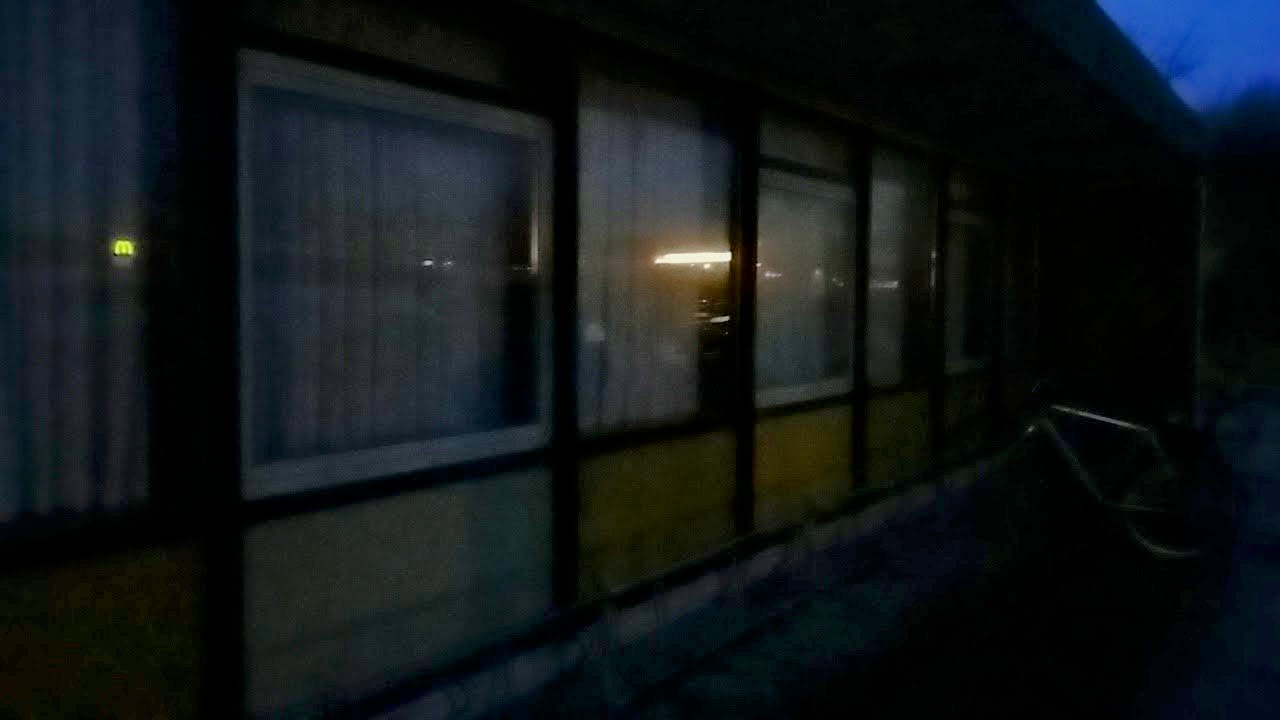This image captures a highly zoomed-in view of the side of a building. In the top right-hand corner, the sky transitions from a dark blue to a shaded area, possibly due to the presence of dark leaves. The extreme zoom makes it difficult to clearly identify objects, but a silver, square-shaped outline is visible on the right side. The left side of the image features a series of windows—four in total—with parts of additional windows appearing along the edges, although they blur into obscurity. Each window is framed in white with a secondary black outline. The building's walls appear to have a yellowish or grayish hue, though the limited lighting makes it challenging to determine the exact color.